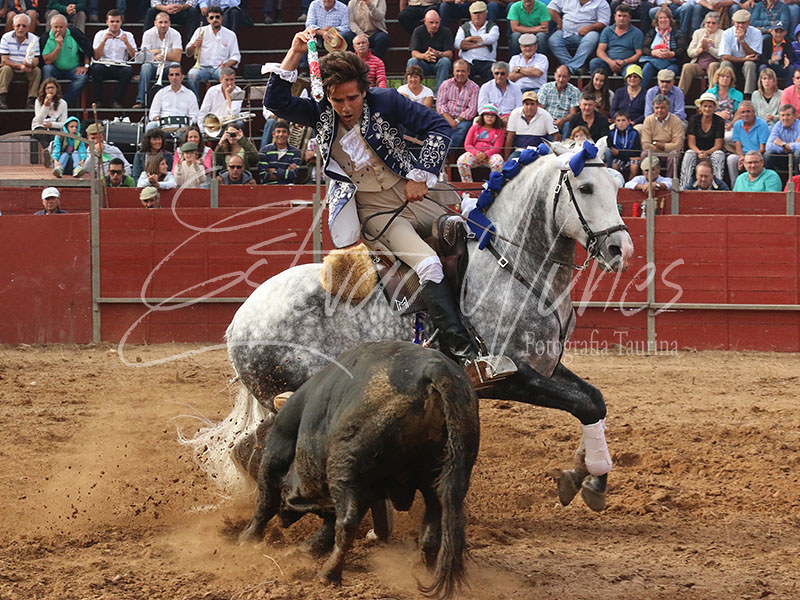The photograph captures a dynamic moment at a rodeo, featuring a man in a regal blue coat reminiscent of an 18th-century suit, complete with a vest, trousers, and black boots. He rides a light grey horse adorned with white spots and blue and white ribbons in its mane. The man is holding the reins in his left hand while his right hand is raised, as if in an attempt to dodge the bull charging towards him. The bull, with its head down, appears aggressive and is heading towards the horse from the foreground. The ground is a soft brown sandy dirt typical of rodeo arenas. In the background, a red wooden fence separates the action from the large crowd of spectators who are intently watching the unfolding scene. The entire setting is bathed in natural daylight, highlighting the vivid colors and intense atmosphere. A watermark, which appears to say "Nunez Fotografia Taurina," is faintly visible over the photo.